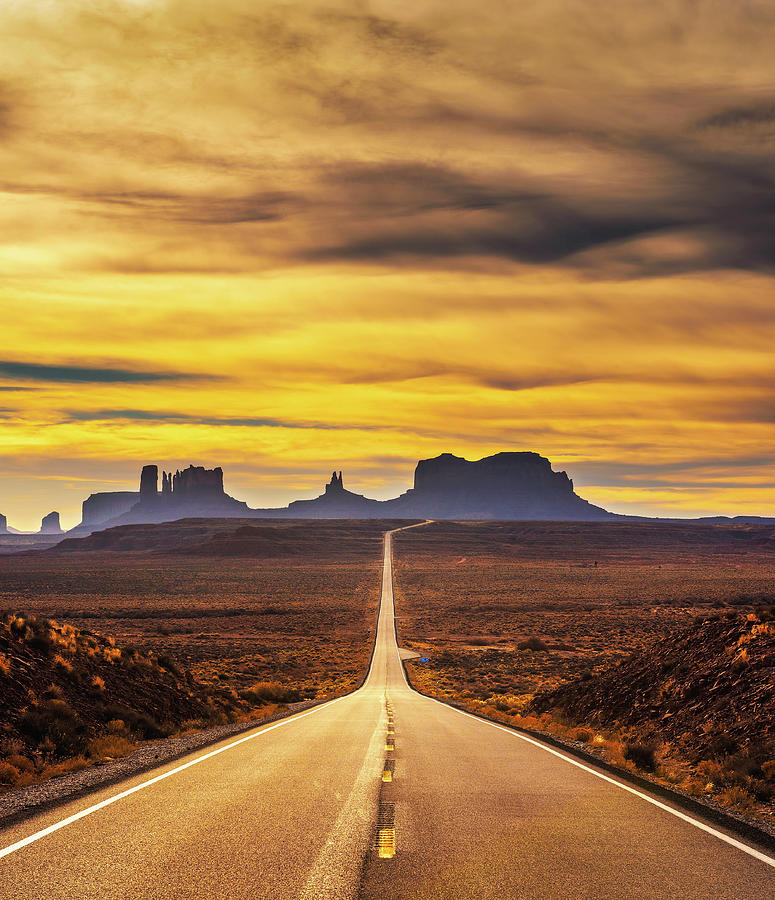The image captures a stunning desert landscape at sunset, featuring a straight, two-lane asphalt highway with yellow dashed lines in the center and white boundary lines, which cuts through the sandy, orange-tinged terrain. The road, which takes up the entire bottom area of the vertical rectangular frame, eventually curves to the right as it narrows into the distance. Gentle inclines of hilly terrain adorned with sparse brush line both sides of the highway, gradually flattening out before rising again into tall, dark rock formations. These formations appear shadowy against a sky painted with vibrant strokes of yellow, orange, gray, and hints of blue and black. This mesmerizing scene is illuminated with a golden hue due to the setting sun, highlighting the dramatic textures and colors of the desert landscape. In the distant background, the road seems to navigate either around or through these towering rock outcroppings, completing the picturesque vista.